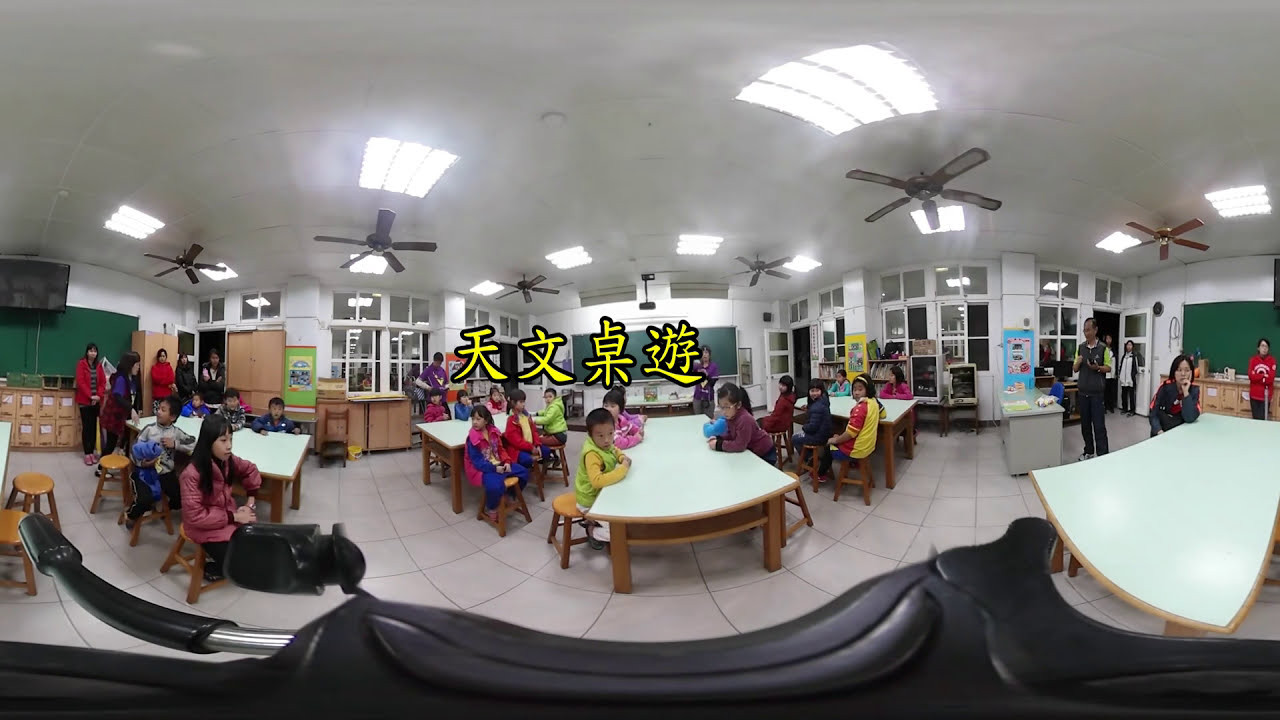This panoramic, 360-degree image captures the interior of what appears to be an Asian classroom, possibly in Japan or China, given the yellow Asian characters displayed prominently in the middle of the image. The fisheye lens effect causes the room to bulge and curve, giving a distorted yet comprehensive view of the entire space. The classroom is bright and orderly, with approximately 20 students seated at several large tables that have white tops and brown wooden legs. The children, who are wearing a variety of bright colors such as yellow, green, orange, red, blue, and pink, are sitting on brown wooden stools. 

The room features a light tan or white ceramic tiled floor and the walls, as well as the ceiling, are painted white, enhancing the brightness of the space. Numerous windows line the walls, and some doors are visible, some of which are open. Ceiling fans and lights are installed overhead, ensuring the room is well-lit. 

A dark green chalkboard is mounted on one of the walls, adding to the academic atmosphere. Towards the sides and near the doors of the classroom, several adults, likely parents or guardians given their neutral-colored attire such as jackets and long-sleeved shirts in red and black, stand observing the scene. The teacher’s desk is positioned to the left, suggesting that this might be a science classroom, and there are stations with books and cupboards along the walls. The absence of natural light implies it might be evening, possibly during a parent-teacher conference or an evening class session.